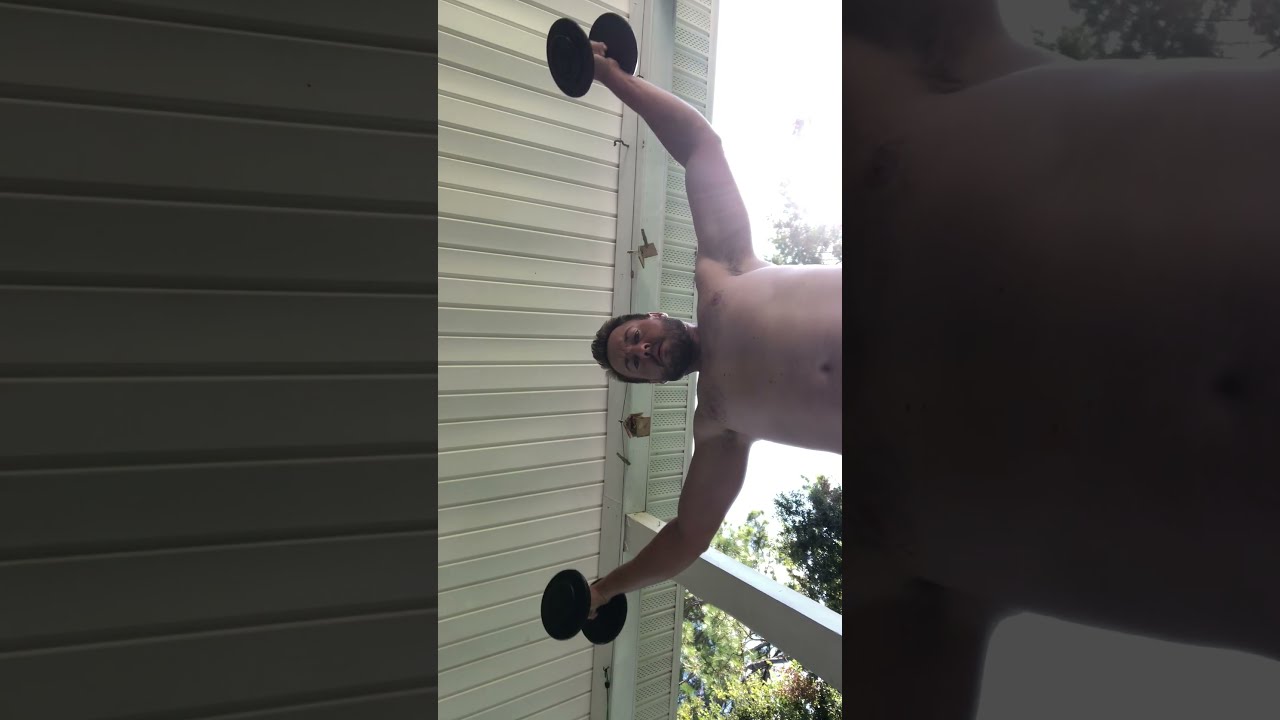The image, presented sideways, depicts a shirtless Caucasian man standing on a porch with short dark hair and a goatee, lifting two black handheld barbells, one in each hand, raised above his head. The porch roof, with its white wooden boards, is supported by at least one large pillar. In the background, the bright sunlight filters through a canopy of trees, highlighting the foliage in a spectrum of light and dark green, creating a vibrant natural setting. While no other people or text is visible, the image's brightness suggests it was taken during daylight hours.